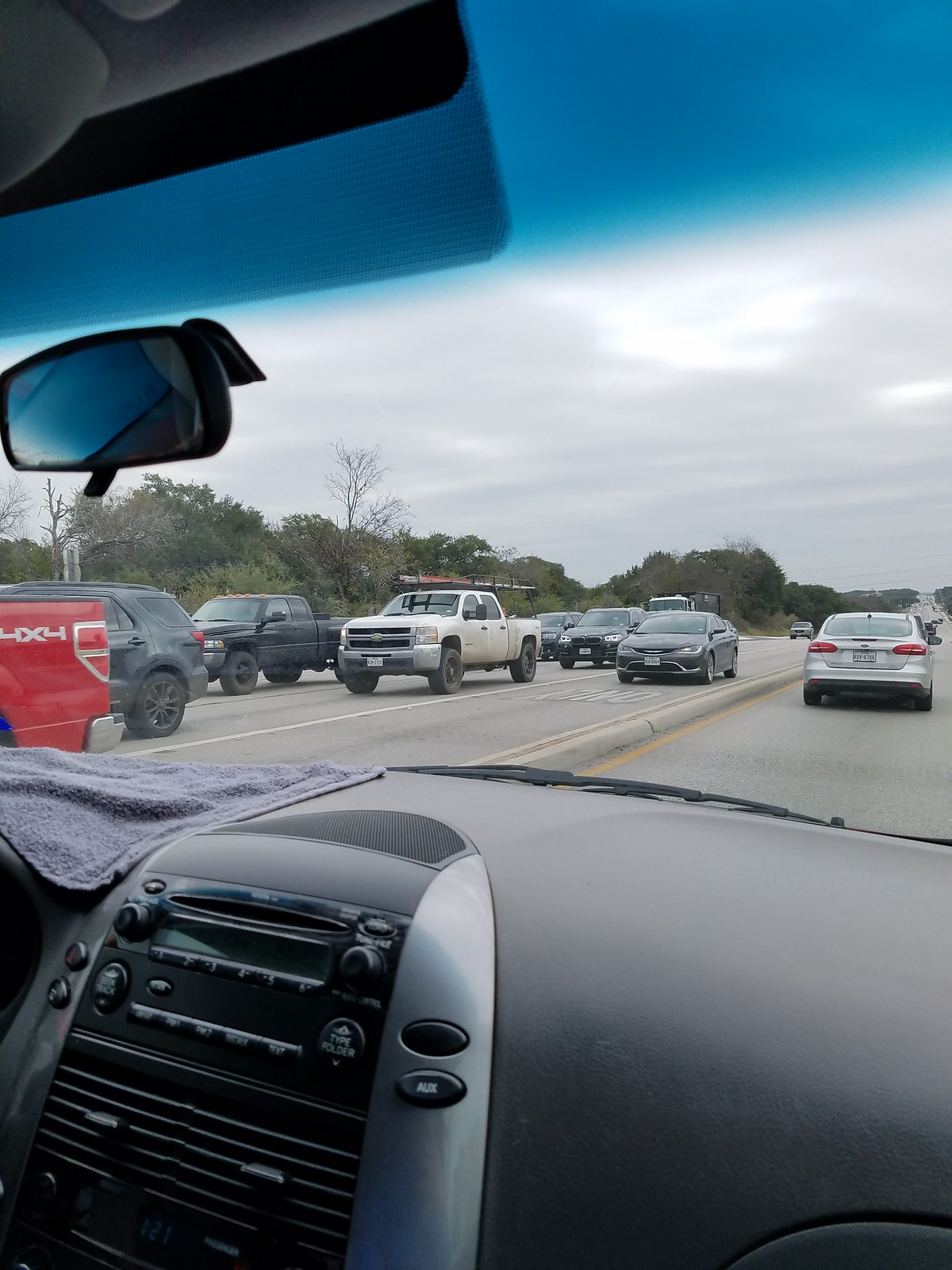The photograph captures a dense traffic jam from within a vehicle. The interior of the car features a black dashboard and a central silver console equipped with a CD player. The console has a screen flanked by two knobs and several buttons below it, along with two larger buttons on the left and right sides, and additional smaller buttons between them. Below the console, there are two air vents with horizontal slats and a small central dial for adjusting airflow. A towel is draped over the left side of the dashboard, and a blue-tinted section is visible at the top of the windshield.

Outside, various vehicles contribute to the traffic congestion, including a white truck, a black truck, a black SUV, a red truck, three black cars, and a silver car. The scene is framed by green trees on the left and a cloudy sky dominated by dark gray clouds above.